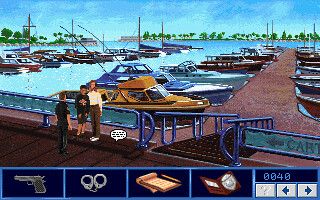In this screenshot from a video game, we witness a serene marina filled with an array of boats. In the foreground, numerous power boats are neatly docked, while in the background, several sailboats rest with their sails down, gently bobbing in the water. The setting creates a picturesque nautical atmosphere, enhanced by the calm, light blue waters and a clear sky.

At the forefront of the scene, three characters stand on the dock, just before a ramp leading to the boat berths. The central figure, facing away from the camera, appears to be a police officer engaged in conversation with two individuals: one clad in a black hoodie and the other in a white shirt. The interaction hints at a possible investigation or routine check.

Overlaying the bottom of the screen is a user interface typical of video games, offering the player interactive options. Icons displayed include a gun, handcuffs, a notepad, and a police badge, suggesting various tools or actions the player can select. In the bottom right corner, the screen displays the numerical code "0040," possibly indicating the player's score or a game-related metric, alongside left and right arrows for navigation.

Overall, the harmonious blend of the marina's tranquil setting and the interactive game elements creates a vivid and intriguing snapshot of the gameplay experience.